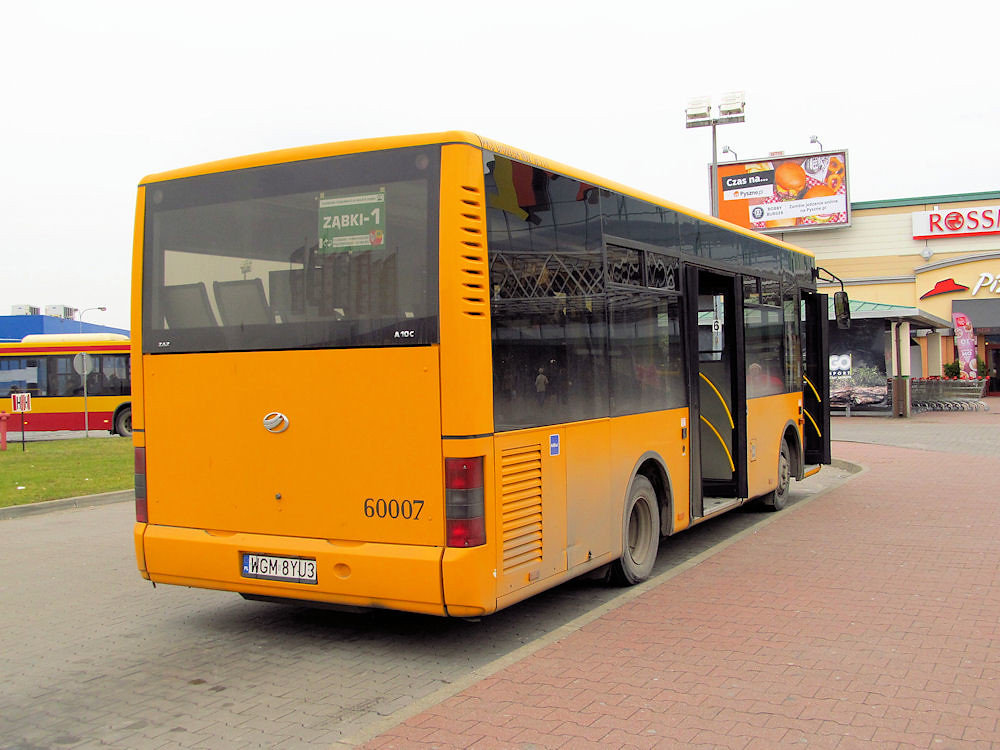The image showcases two buses parked along a walkway in front of a shopping center. The prominent bus in the foreground is a vibrant yellow with dusty tires and black-tinted windows that stretch from the midpoint to the roof. The bus is labeled with the number "60007" on the rear and has a green sign in the back window reading "ZA8KI-1." The bus's front and middle doors are open, revealing yellow railings and a bit of the interior seating.

The pavement on which the bus is parked is made of beige-colored brick, while the adjacent sidewalk consists of red bricks arranged in a similar pattern. Behind this bus, partially obscured, another yellow bus with red and yellow stripes is visible near the left side of the image.

In the background, a beige building with white and green trim hosts a sign that reads "ROSS" in red letters. Below this sign is the recognizable logo of Pizza Hut. Additionally, a taller sign featuring a picture of a hamburger and french fries is visible, and a streetlight is mounted nearby. The entire scene is bathed in daylight, with a clear, almost white, blue sky encompassing the area.